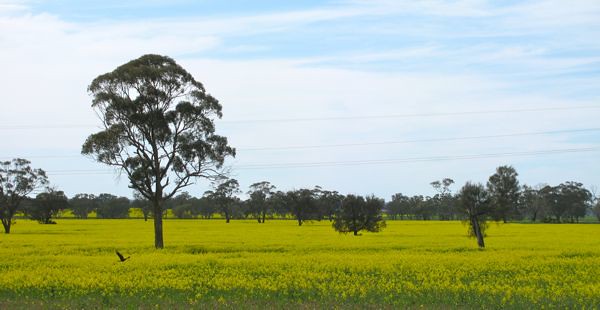The image captures a lush grassy field under a bright blue sky that is scattered with wispy white clouds. The ground is dotted with greenish-yellow grass and bushes, adding a touch of vibrancy to the scene. Trees, possibly some kind of fir, are sporadically spread across the landscape; in the foreground, there is a noticeable larger tree positioned towards the left third of the image. These trees have minimal foliage, contrasting with more densely packed trees further in the background. Subtle power lines, barely discernible, stretch across the sky from left to right. A bird, appearing brown, is flying from left to right, adding a dynamic element to the serene countryside setting. The photograph, likely taken during daytime, showcases an open field evocative of a farm or rural environment.